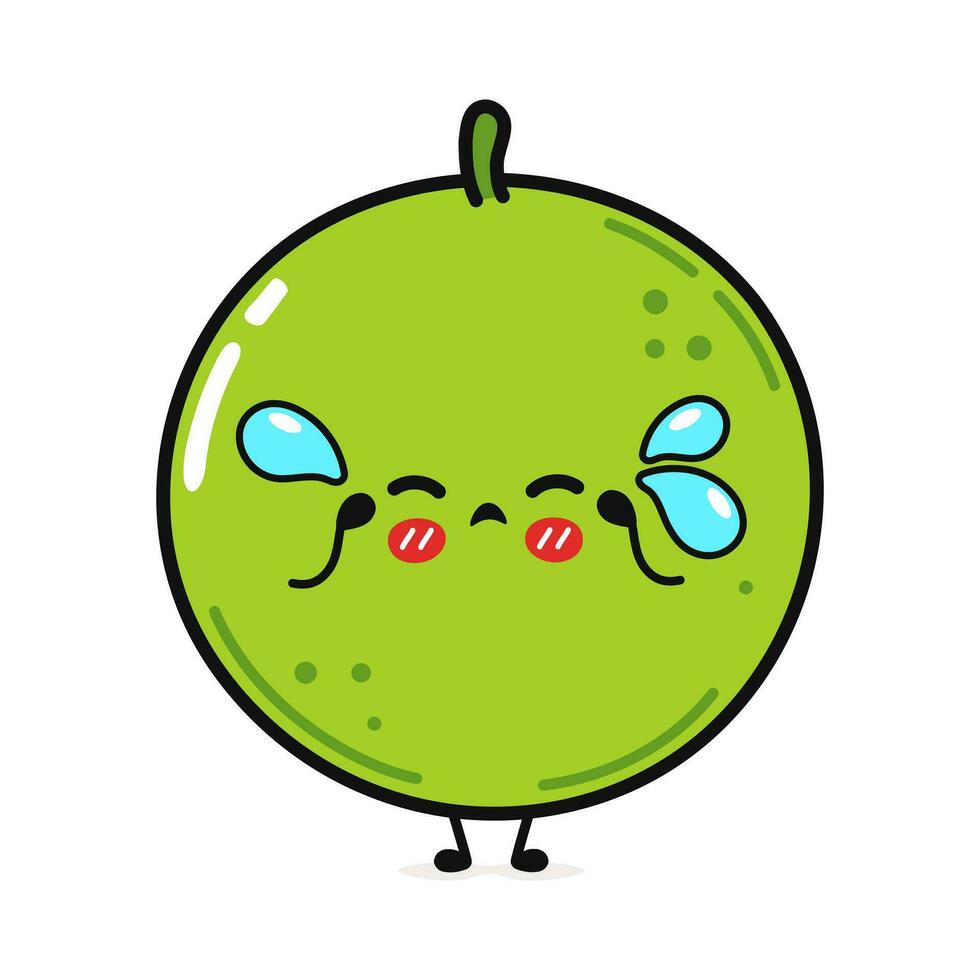The image features a digitally drawn character that resembles a lime green apple or possibly a lime, characterized by its round, circular shape with a small, dark green stem protruding from the top. The apple-like figure has a black outline accentuating its form, also containing segments with darker green hues. The face centered on the circular shape includes closed squiggly lines representing the eyes, from which three blue tears appear to be falling—two from the right eye and one from the left. Its small, rosy-red cheeks and tiny black nose add to the expressive visage. The character also has two black arms positioned near its eyes, giving the impression it is rubbing them, further emphasizing the crying expression. Completing the image are two black, music-note shaped feet at the bottom, and a few sporadic greenish lines and dots around the object, with a hint of white glare on the left side reflecting light. The entire composition sits against a plain white background.